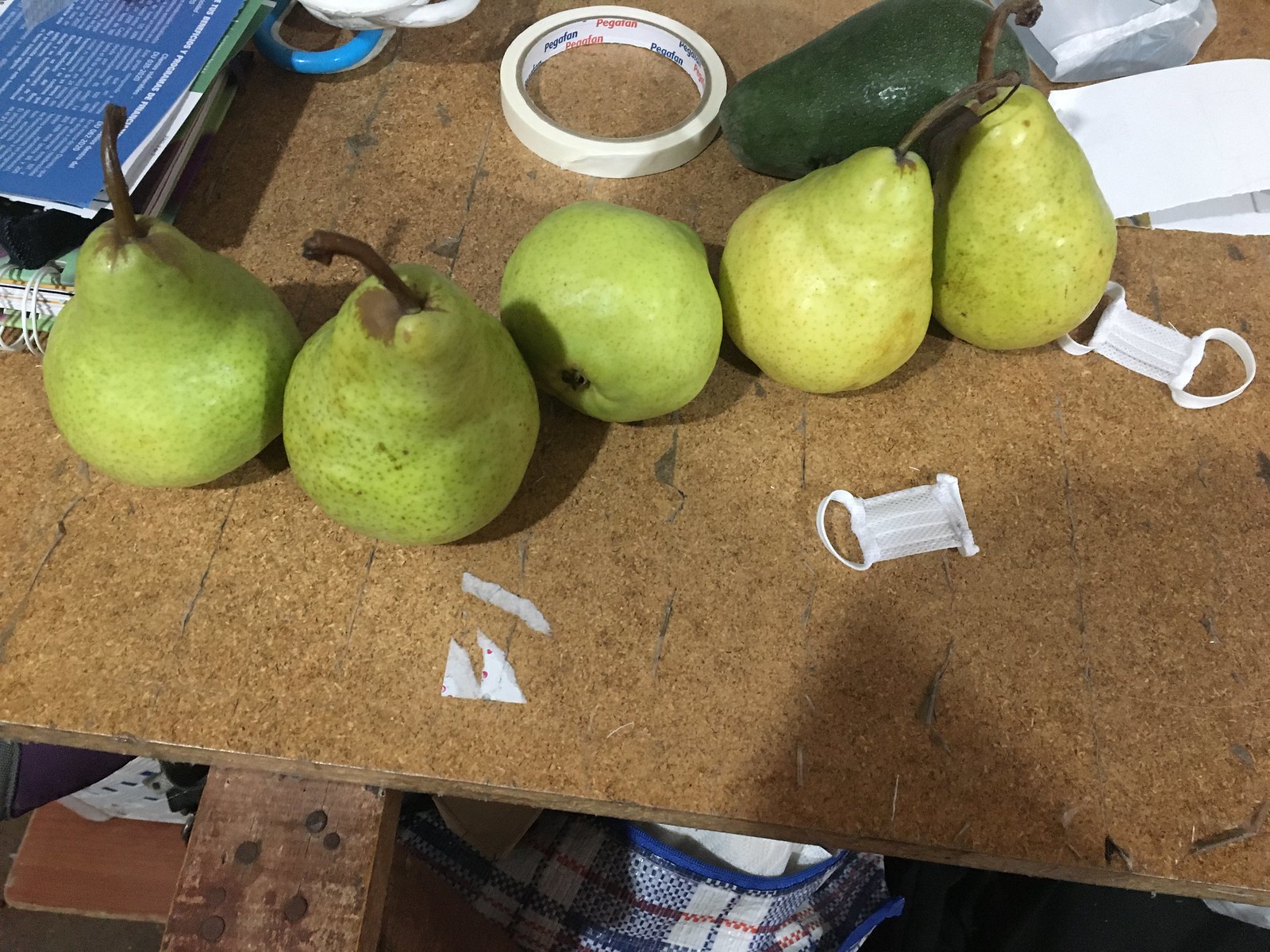The image is a digital photograph likely taken outdoors, judging by the natural lighting and reflections. The main focus is a light tan wooden table with five pears scattered across it. These yellowish-green pears, some with brown spots, vary in position—some standing upright and others knocked over. In the upper left corner, there’s a blue book with white, illegible writing next to several coat hangers, predominantly white, except for one blue hanger. Nearby is a roll of white masking tape, and alongside it, a very dark green fruit, possibly an avocado, is visible. In the upper right corner, two white paper bags are present. A white medical mask lies adjacent to the rightmost pear, and another mask is situated slightly left and more towards the front. Underneath the table, a mostly white checkered bag with blue stripes is noticeable. Additionally, scattered around the wooden surface are rubber band fasteners, contributing to the cluttered scene that appears to be in a garage or workshop setting. The shadow of the person taking the photo can also be seen, adding to the composition’s context and dynamism.